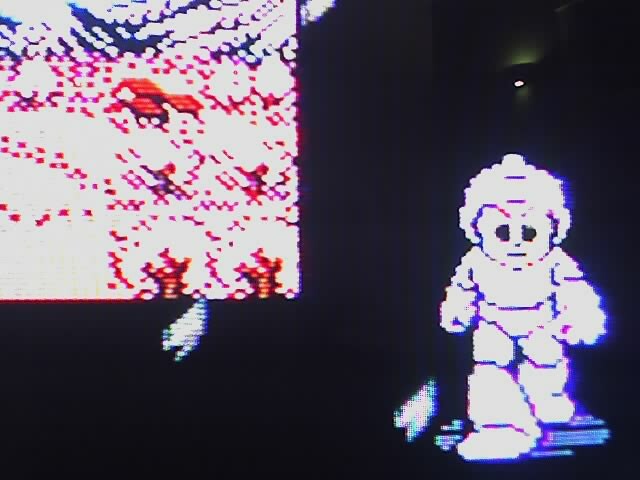In this image, a video game character is depicted with a distinct yet familiar design. Positioned on the left side, the character is primarily white with dark lines outlining the segments of his body and legs, reminiscent of the Michelin Man. The figure has a robotic appearance, suggesting he might be in some kind of space suit, highlighted by a human-like face. The image is mostly dominated by dark tones, adding to the mysterious ambiance.

Above the character on the left, there is a small source of light that appears to be from a room, enhancing the illusion that this character is transitioning from a digital to a real-world environment. On the right side, a large pixelated square adds to the surreal atmosphere with a mix of white, red, blue, and purple hues. Within this colorful and chaotic square, there appear to be elements resembling a house with red roofs, all swirling together in a blend of reds, pinks, purples, and blues.

Despite the dark and complex background, the character's simplistic and bold design stands out, making him the focal point and hinting at his significance in the narrative, even if his exact origins remain unclear.